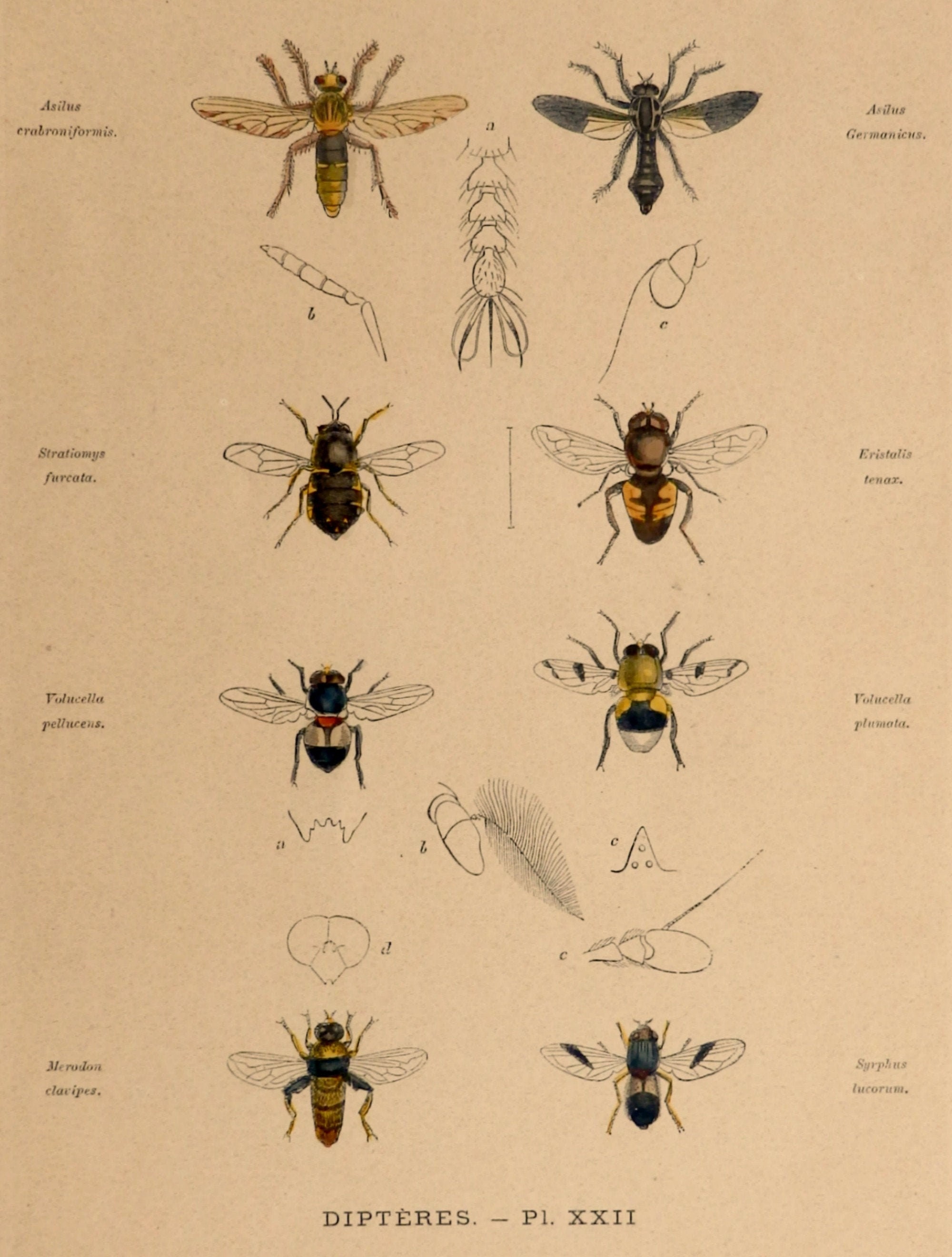The image appears to be a yellowed page from a professional entomological book, featuring hand-drawn and hand-painted illustrations of eight different types of winged insects, arranged in two columns of four. The background is an off-white color, and the text, while too small to read clearly, includes the scientific names of the insects on the left and right edges, with names like Acillus araboniformis and Anilus germanicus being discernible. The insects predominantly appear to be various types of flies and bees, each depicted in vivid colors including black, white, gray, yellow, blue, red, and green. The detailed illustrations show the insects with beady eyes and typically six legs, although some may appear to have four. Additional black outlines highlight and label specific body parts. The top two insects are slender, with one being yellow and the other black and white. Further down, there are stouter insects with one black and yellow, another brown and orange, followed by a blue-red-silver one and a golden-blue-silver one. The final row features a green-yellow insect and a blue-white insect. The bottom of the page is annotated with "dipterus-pixx11."